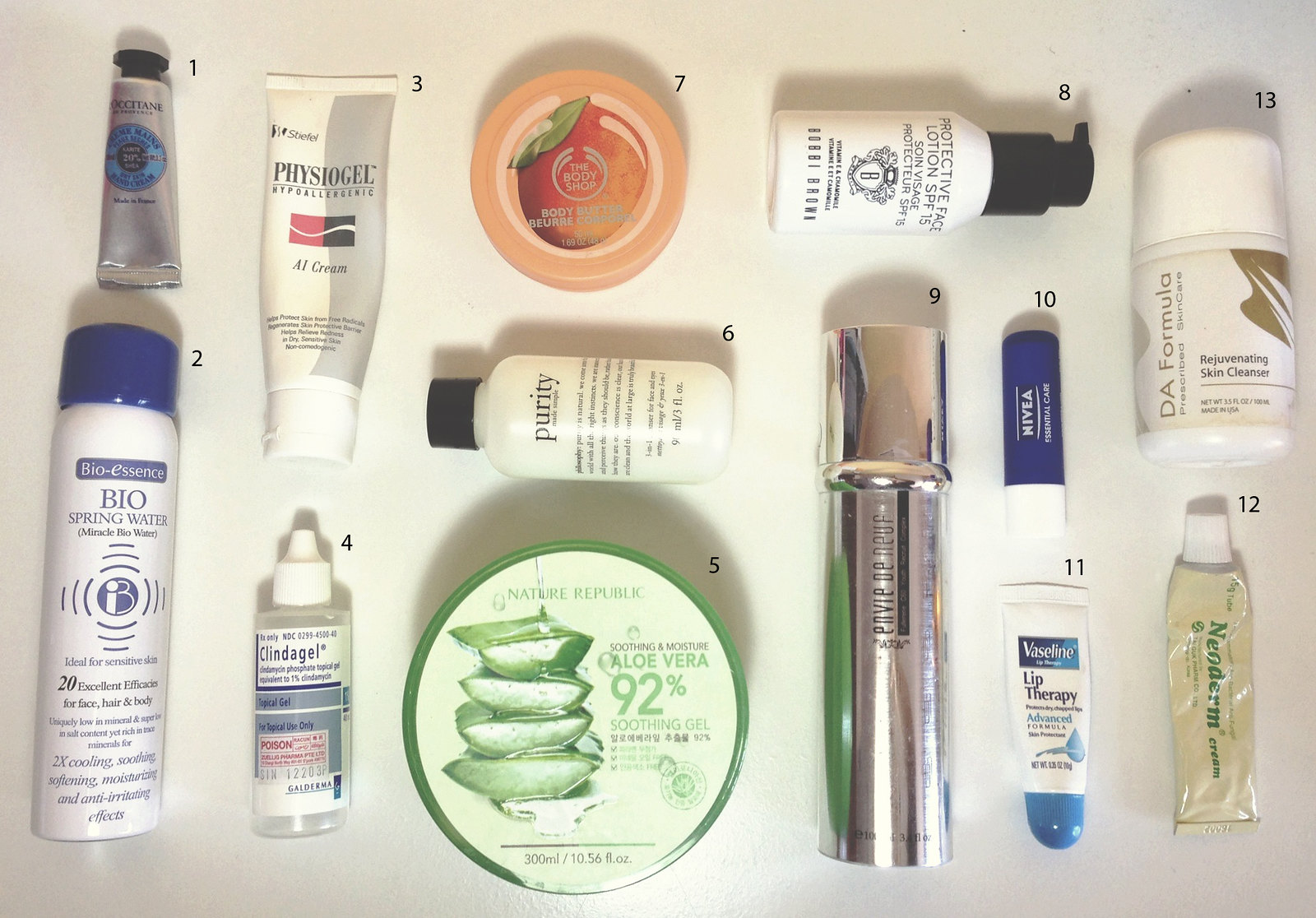This meticulously staged photograph showcases an array of 12 diverse beauty products, all strategically lined up against a pristine white backdrop, illuminated by a soft light from above. Each product is numbered, creating a sense of organized presentation and emphasizing their distinct qualities.

1. **L'Occitane Hand Cream**: The first product is a small tube of L'Occitane lotion, characterized by its sleek, compact design, though the exact label details are somewhat indiscernible.
2. **Physiogel Cream**: Following is a white tube with a matching cap, containing Physiogel cream, known for its moisturizing properties.
3. **Body Shop Body Lotion**: Next in line is a container from The Body Shop, potentially offering a delightful peach scent based on its label.
4. **Bobbi Brown Face SPF**: This item is presented in a chic black and white pump bottle, ensuring convenient application of Bobbi Brown's facial sun protection formula.
5. **DA Formula Rejuvenating Skin Cleanser**: Highlighted in an elegant gold and white bottle, this cleanser promises a revitalizing skin routine.
6. **Lip Therapies Cluster**: In the bottom right corner, there is a charming cluster of various lip therapy products, catering to different lip care needs.
7-12. **Assorted Face Washes and Lotions**: The remainder of the lineup includes an assortment of face washes and lotions, completing the comprehensive collection.

This curated assembly not only highlights the diversity in skincare and beauty products but also reflects a meticulous effort in their presentation, aimed at drawing the viewer’s attention to each individual item within the ensemble.